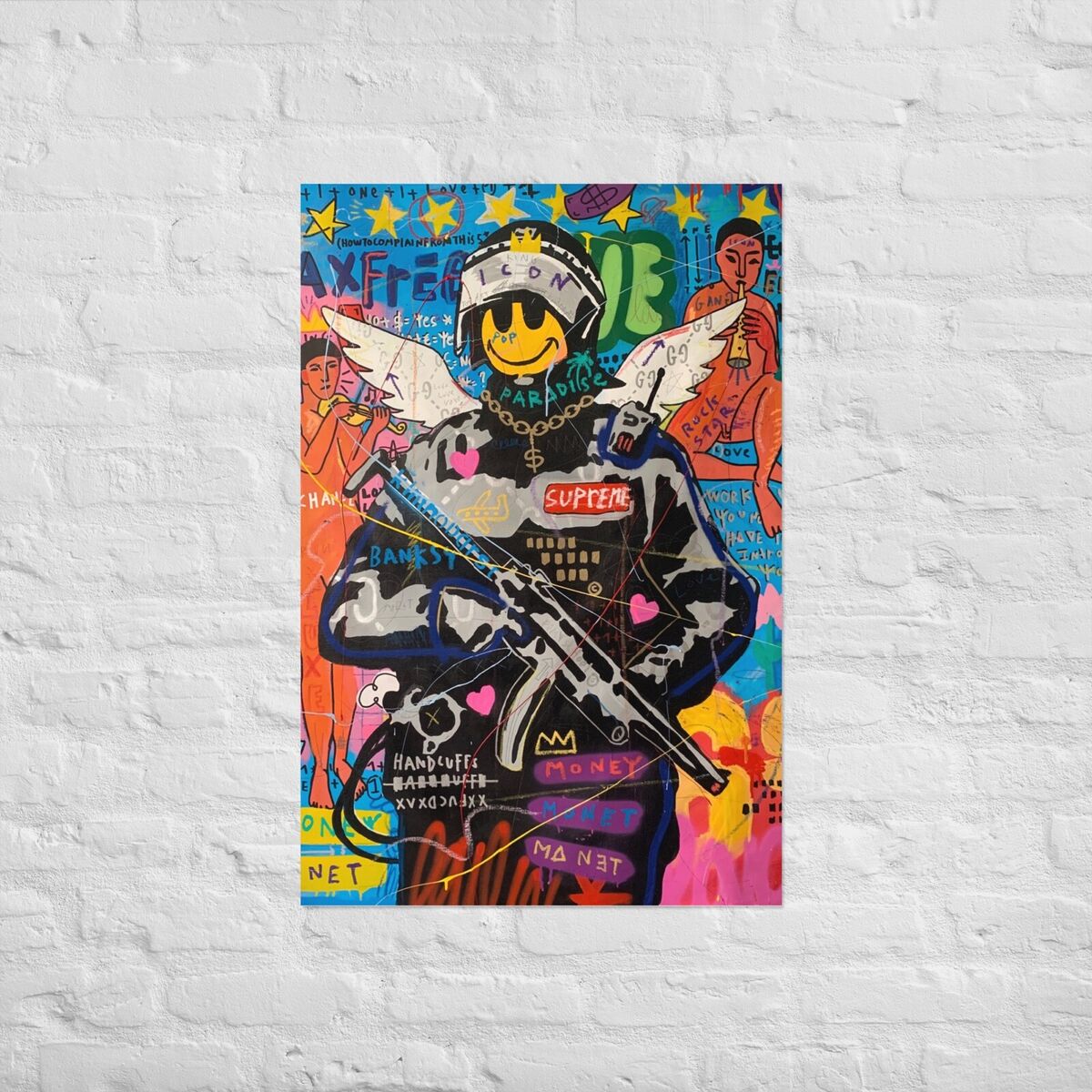The poster, centrally displayed on a white-painted brick wall, commands attention with its vivid, eclectic mix of imagery and color. Dominated by a drawing of a smiley face, which serves as the face of a figure adorned in black and gray military attire, the image is loaded with symbolic elements. This figure is holding an automatic rifle aimed towards the bottom right and is accessorized with a gold necklace, police helmet, and white angel wings sprouting from its back. The collage-like composition includes an array of vibrant hues—pink, red, yellow, and more—creating a visually stimulating effect. Yellow stars line the top of the poster, while other motifs such as pink hearts, a small crown with the word "money" beneath it, and possibly branded names like Supreme add layers of cultural commentary. In the upper right, there's a smaller figure playing an instrument, adding to the chaotic yet intriguing mix of elements. The overall aesthetic is graffiti-esque and cartoonish, evoking a contemporary artistic style that might be attributed to notable street artists, possibly even Banksy.